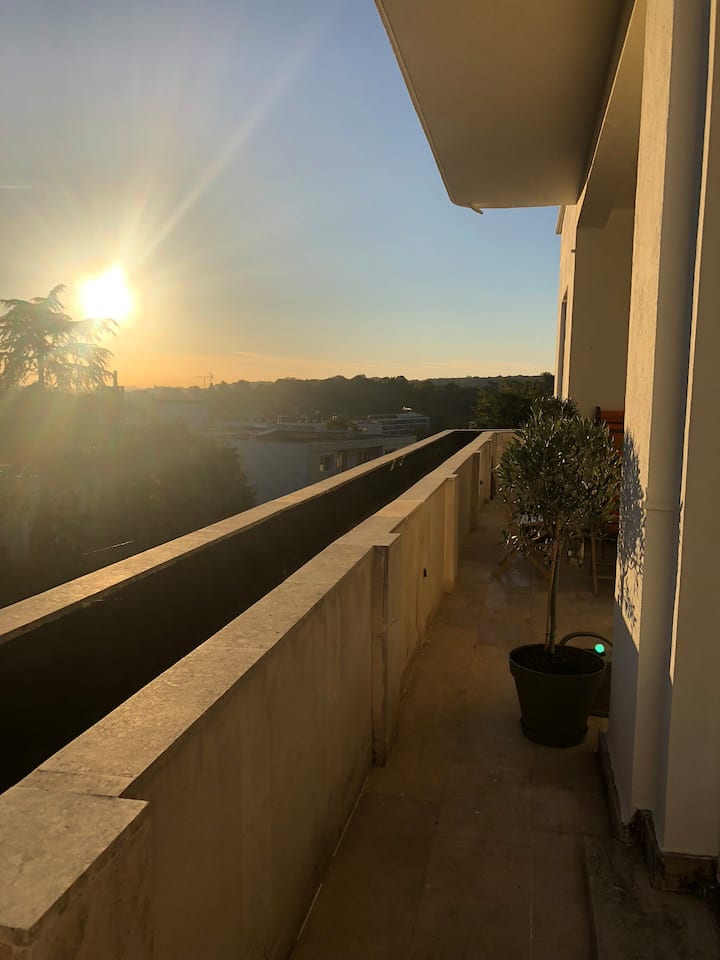The image depicts a long, narrow balcony made of light beige brick or tan concrete, adorned with a smooth concrete railing on the left. A slender potted tree with green leaves stands on the balcony in a black pot. The building hosting the balcony features an overhang, likely part of another balcony or roof. Sunlight shines over the horizon, casting beams upward and illuminating the vivid blue sky with golden hues near the edges. In the background, lush green trees contrast with the sky, while further below, additional buildings and trees are visible. The scene, devoid of any people, captures the tranquil beauty of nature meeting urban living.